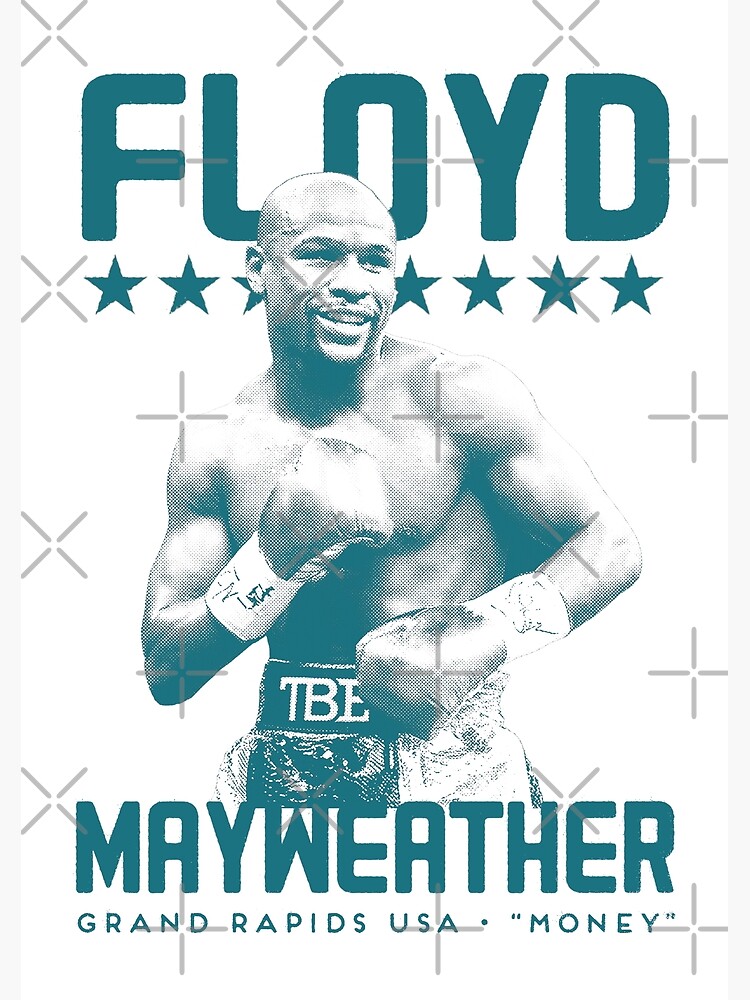This poster features the renowned boxer Floyd Mayweather, depicted in a detailed pen and ink drawing. He stands at the center of the image, shirtless, wearing his boxing trunks emblazoned with the initials "TBE" and boxing gloves, ready to fight. Mayweather's face bears a confident smile as he looks to his left. The poster employs a muted palette of grayish-white and dark teal blue colors, adding a sophisticated, vintage feel. The background is white, adorned with decorative gray X's and plus signs that span the poster, including over the text and image.

At the top of the poster, in large, bold dark teal blue letters, is "Floyd," accompanied by a series of solid blue stars directly underneath. Midway down the poster, there is the illustration of Floyd Mayweather himself, his determined stance suggesting readiness. Below his image, the text "Mayweather" appears prominently, followed by "Grand Rapids USA" in smaller letters. At the bottom right, the nickname "Money" is featured in quotation marks, encapsulating his famous moniker. This evocative poster captures the essence of Floyd Mayweather as a formidable and celebrated figure in the boxing world.